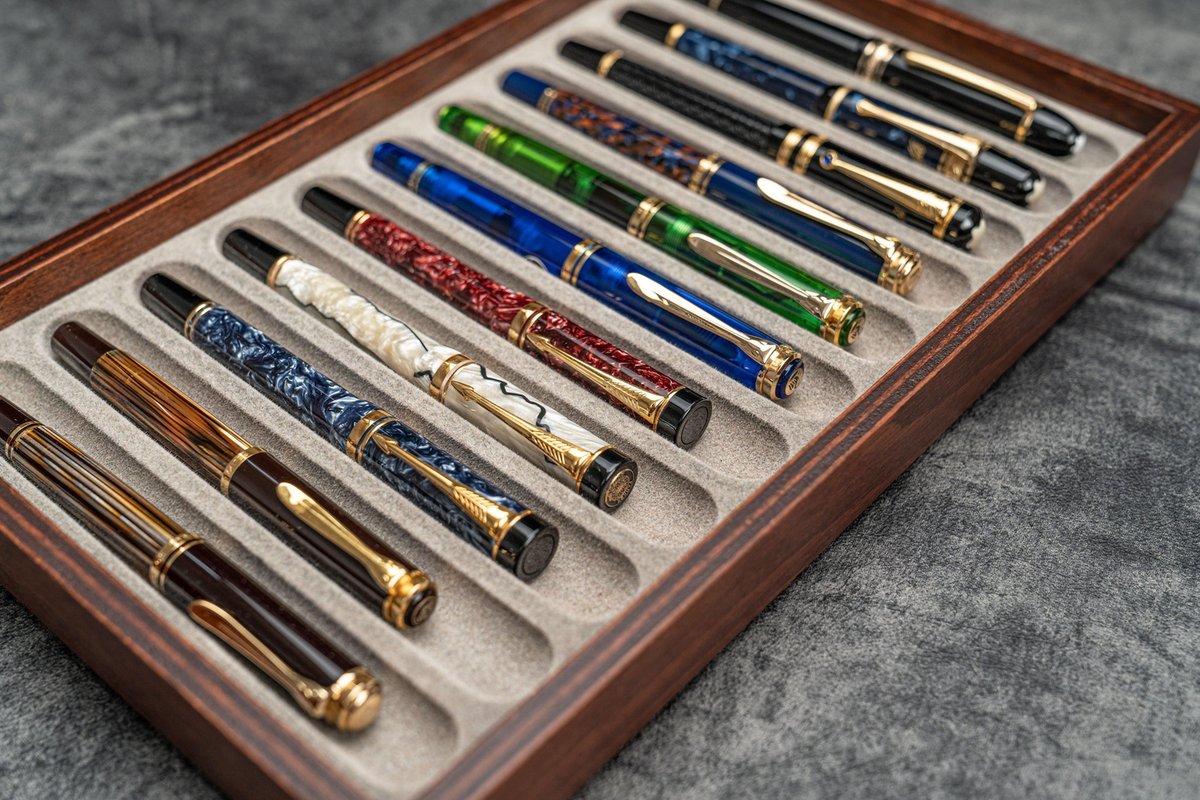The image showcases an artistic, horizontally rectangular photograph taken indoors, featuring a high-quality stained wooden display case. The background consists of a textured grey, white, and black countertop, devoid of any border. Inside the display case, there are 11 individual slots, each holding an elegantly designed, high-end fountain pen. These pens require the cap to be pulled off to access the writing tip. The collection boasts an array of colors and designs, including beautiful wood finishes, striking reds, various shades of blue, green, black, and an ivory-colored pen with additional decorations. Each pen is equipped with a clip, emphasizing their premium quality and sophisticated aesthetics. The pens are elaborately crafted and intended for luxurious use, distinguishing them from ordinary writing instruments.